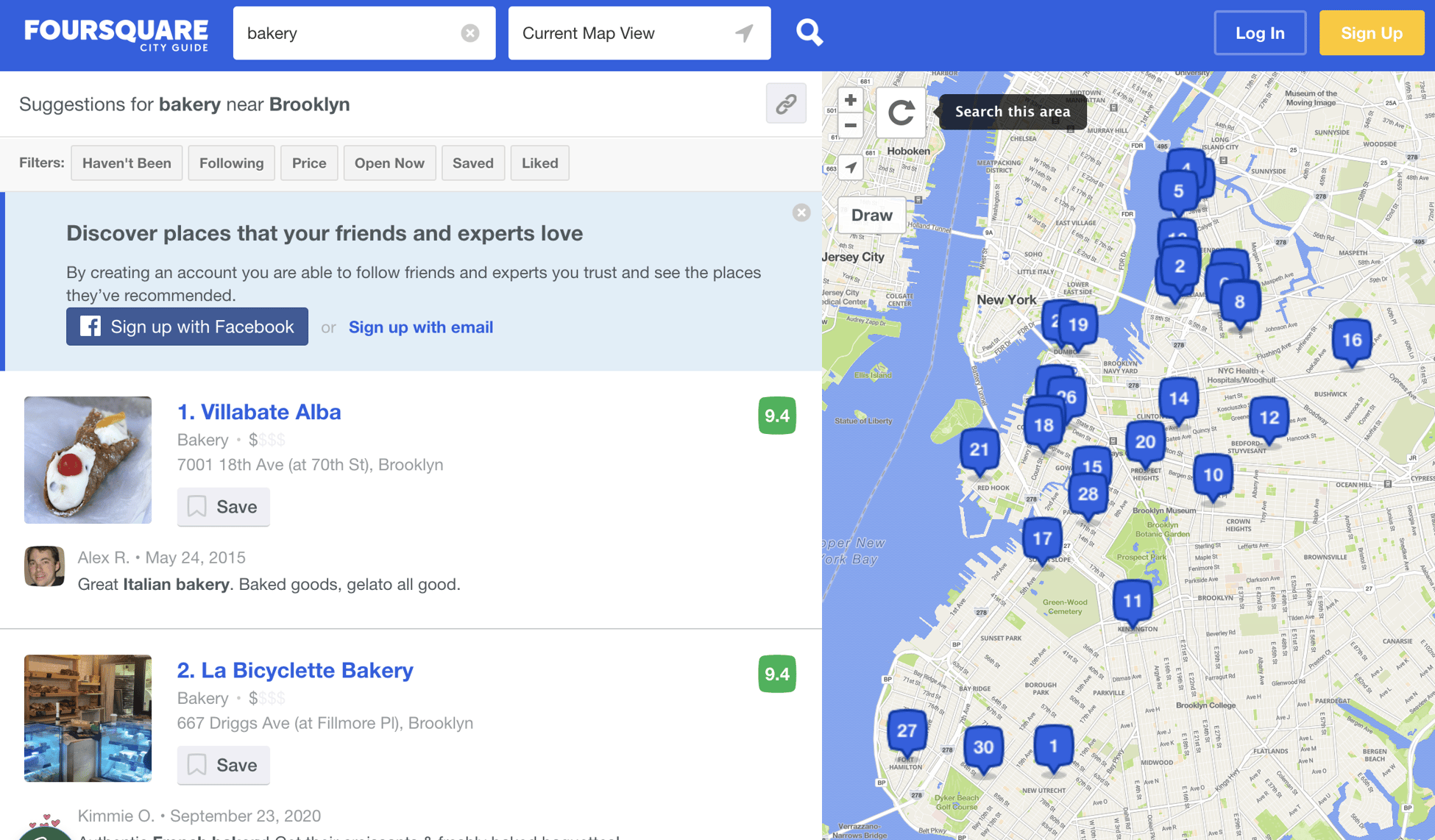The image displays a Foursquare website interface with a top blue banner featuring prominently the white, all-caps text "FOURSQUARE." Directly beneath this, in a refined all-caps style, is the text "CITYGUIDE." Below the banner is a search bar with the term "BAKERY" entered, next to an option labeled "CURRENT MAP VIEW." Additionally, adjacent to the blue banner is a white magnifying glass icon and text prompting users to "LOG IN AND SIGN UP," with "SIGN UP" highlighted on a yellow background.

Progressing down the page, a white background section displays the text "SUGGESTIONS FOR BAKERY NEAR BROOKLYN." Further down, a light gray banner provides filter options labeled "Haven't Been," "Following," "Price," "Open Now," "Saved," and "Liked." Another section of the blue banner encourages users to "DISCOVER PLACES THAT YOUR FRIENDS AND EXPERTS LOVE," providing options to "SIGN UP WITH FACEBOOK" or "SIGN UP WITH EMAIL."

Below this, two bakery recommendations are listed: 
1. "Elevate Alba Bakery," described as a "Great Italian Bakery" offering "Baked Goods, Gelato, All Good."
2. "Bicyclette Bakery," with corresponding address details provided.

The right side of the page features a map of the Brooklyn area, with various numbered markers indicating the locations of these and possibly other points of interest.